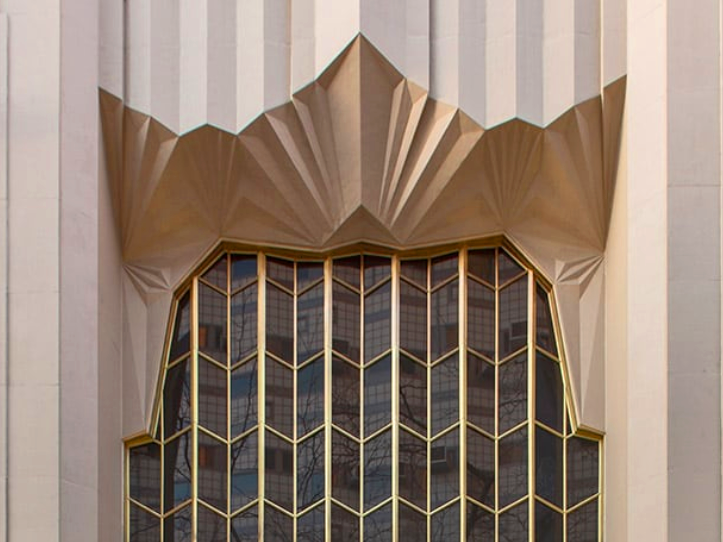The image is a color photograph in landscape orientation, capturing a detailed view of the Art Deco architecture of the Stella Tower Residences in Hell's Kitchen. The central focus is a decorated window framed by geometric gold designs. Above the window is a prominent Art Deco awning that resembles a golden, crown-like structure with three triangular peaks—a large central peak flanked by smaller ones on each side. The building’s facade features a vertical pattern of 45-degree angled squares and rectangles, creating an accordion-like effect. The windows, which are beige with a slight purple tinge, are divided by gold frames and reflect nearby buildings with square windows and some trees. The photograph emphasizes the intricate geometric patterns and rich textures, typical of the Art Deco style.